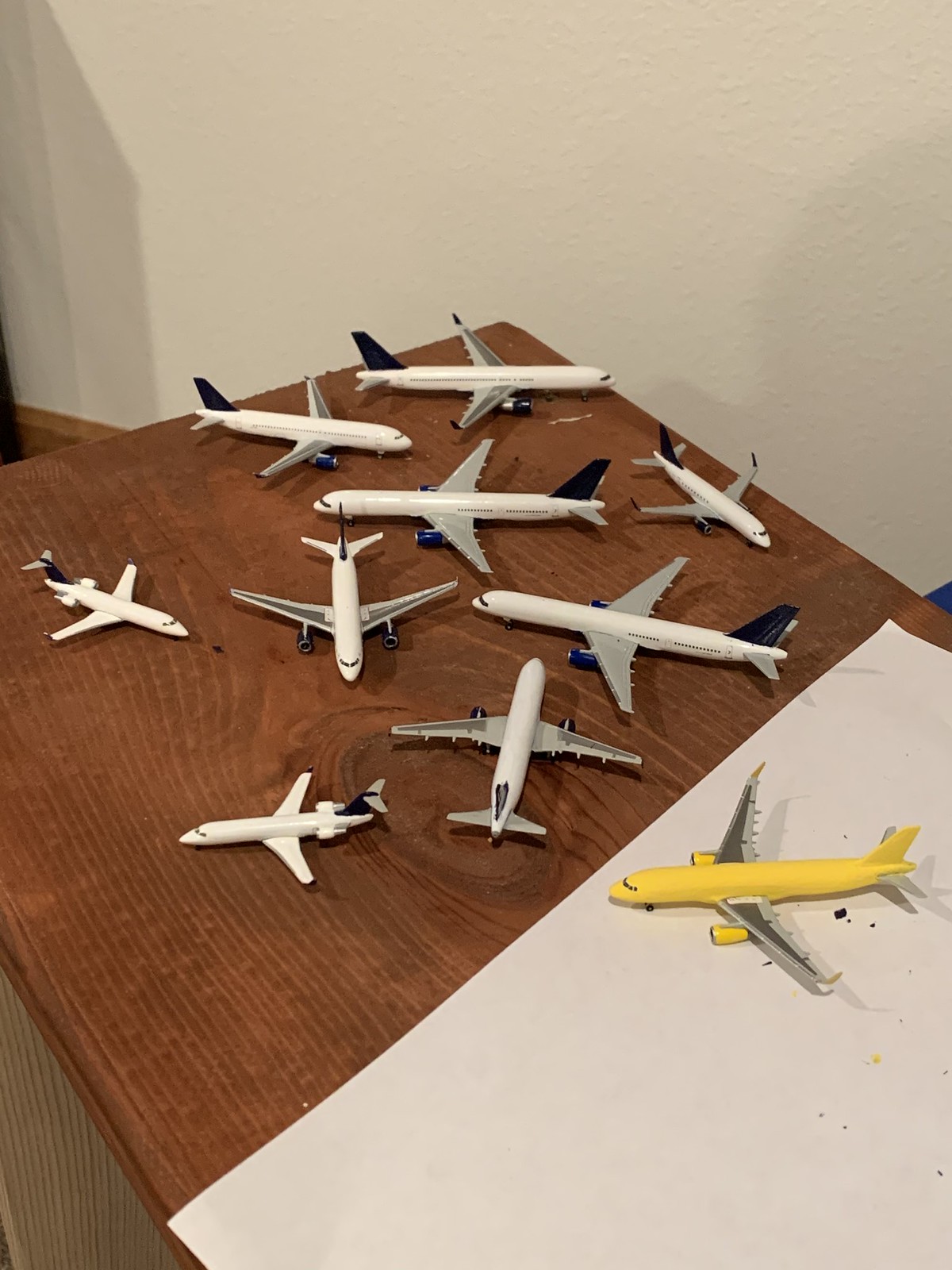This image captures a detailed scene inside what appears to be a hobby or bedroom. Dominating the bottom half of the photo is a wooden table, brown in color, littered with an array of small airplane replicas. To the bottom right of the table, a white sheet of paper or poster board occupies about 30% of the table's surface. On this sheet rests a yellow airplane model with silver and gray wings, positioned to face the left. Scattered across the rest of the table are nine other airplane models, distinguished by their white bodies and blue wings or tails. These models vary in size and are oriented in multiple directions: left, right, up, and down. Two of the planes on the left side of the table particularly stand out, with one headed left and another southeast. The background of the image reveals a white drywall, with a patch of brown boarding visible at the top left corner, suggesting a cozy room dedicated to model building or aviation.